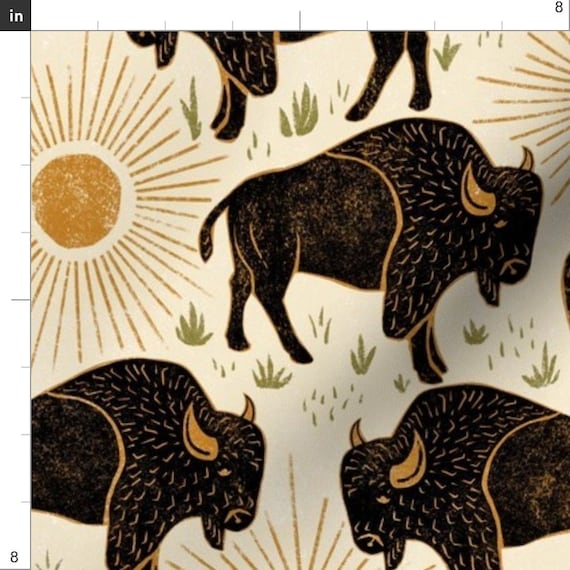This image depicts a computer-generated rendition of Brahma bulls, characterized by a minimalistic yet detailed artistic style. The background is an ivory off-white interspersed with green elements suggesting leaves and trees, further enriched by multiple sunbursts. The most prominent sunburst has a gold center surrounded by a white ring, with gold rays of varying lengths extending outward.

At the center of the image, a fully visible bull displays a striking combination of black and blue fur interspersed with white, and is accentuated by golden horns with black stripes, which add a three-dimensional effect. The bull's face features additional golden accents around the nose and eyes. The thicker fur along the bull's back is distinguished by golden outlines and lines, enhancing its texture.

Surrounding the central bull are glimpses of three additional bulls, each partially cut off by the edges of the image. These bulls share the same intricate detailing, including golden horns, black fur with golden lines, and golden accents. Olive green leaves and tufts of gray-green grass are scattered below the bulls, contributing to the naturalistic yet stylized theme of the composition.